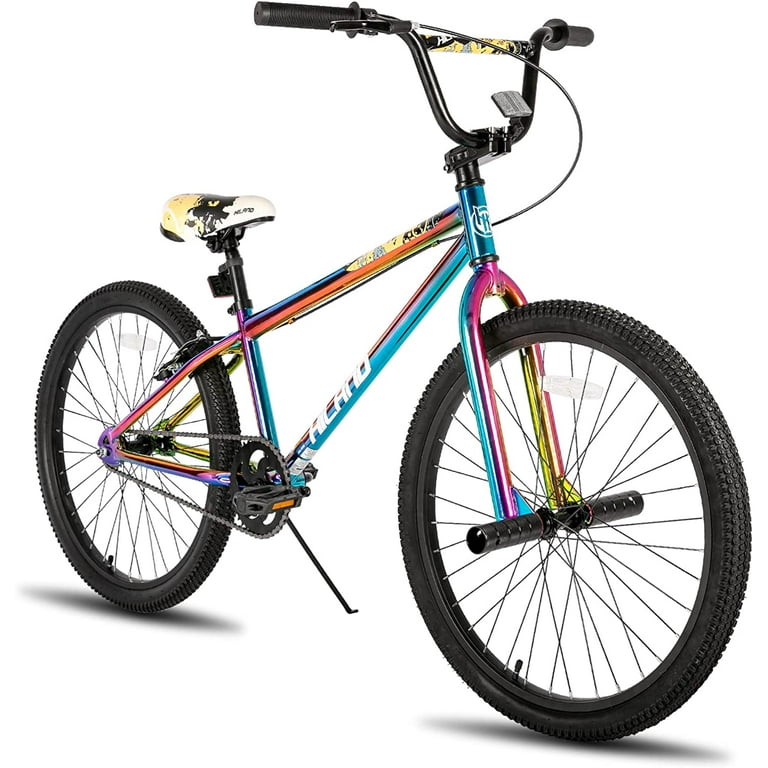This is a detailed image of a vibrant, multi-colored children's bicycle set against a striking red background, prominently featured in a digital advertisement. The bicycle showcases an array of colors and distinctive features: the frame slants are turquoise, with parts blending into blue, purple, orange, and pink near the gears. The lower slant bar is decorated in blue with a purple stripe, matching the fork's pattern. The upper frame transitions from orange and blue to purple at the rear sprocket. The bicycle boasts foot pegs on the front axle, indicative of a design for performing stunts. The chain and gear system are predominantly dark gray, while the kickstand and tires are black. The handlebars and brake bar are black, with rubber grips in matching color, complemented by a headlamp for visibility. The crossbar is multi-colored with yellow, black, and white accents. The seat cushion is a mix of white, black, and yellow leather, featuring a distinctive yellow line pattern. Additionally, the bike includes a reflector on the front. The brand name banner is visible, though somewhat unclear, adding a touch of authenticity to the promotional image.